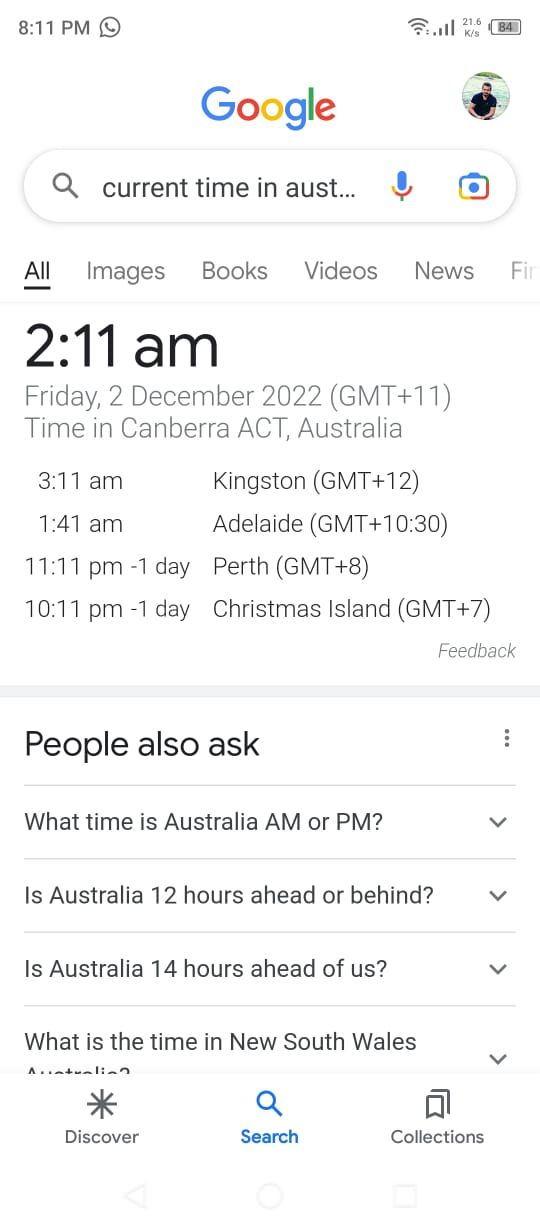This is a detailed screenshot from a mobile phone. The upper left corner of the display features a white background that highlights the current time, 8:11 p.m., in a black font. Adjacent to the time is an icon depicting a chat bubble with a phone inside it, signifying messaging or call notifications. To the right of this icon are indicators for Wi-Fi and mobile signal strength, both showing full bars. The battery level icon indicates an 84% charge.

Directly below this status bar is the Google search bar. On the left side of the search bar is the Google icon, while on the right side is the user's Google account profile picture. The profile picture belongs to a Caucasian male in his 20s, who is seated on a beach wearing a black polo shirt.

Beneath the profile picture, within the Google search bar, there's a typed query: "current time in AUST...". Accompanying the search bar are icons for voice search (microphone) and Google Lens (camera).

Below the search field is a horizontal navigation menu offering search result categories: "All," "Images," "Books," "Videos," "News," and "Fi...".

Displayed prominently in bold black font is the local time result: "2:11 a.m." Under this, in gray font, it states "February 2 December 2022 GMT+11 - Time in Canberra, ACT, Australia." Additional times for other locations around Australia are listed as follows:
- Kingston: 3:11 a.m. GMT+12
- Adelaide: 1:41 a.m. GMT+10:30
- Perth: 11:11 p.m. one day prior, GMT+8
- Christmas Island: 10:11 p.m. one day prior, GMT+7